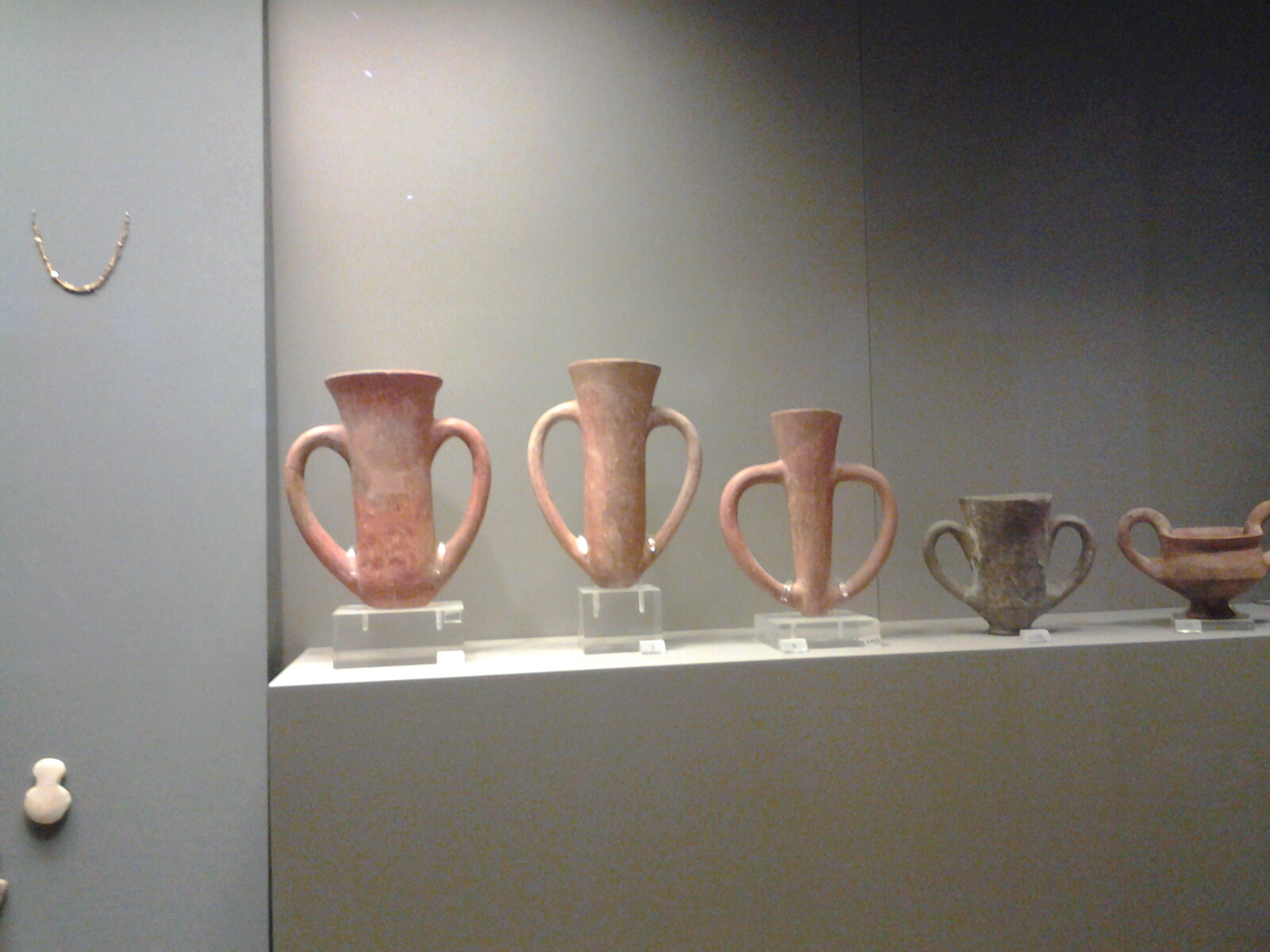The image depicts a dimly-lit photograph taken inside a museum, featuring a carefully arranged display of five vases on a white table with a brown base, set against a corner where a white wall meets a blue one. The vases vary in size and color; some are tall and rose-colored while one is flatter and grayish-green. Each vase has notably wide handles, suggesting an ancient, possibly clay-crafted origin. Adjacent to the table are other artifacts, including a necklace hanging on the wall. The scene is captured through a grainy lens, hinting at low lighting conditions within the gallery space. The vases are placed on clear acrylic stands, enhancing their prominence and visibility in the exhibit.